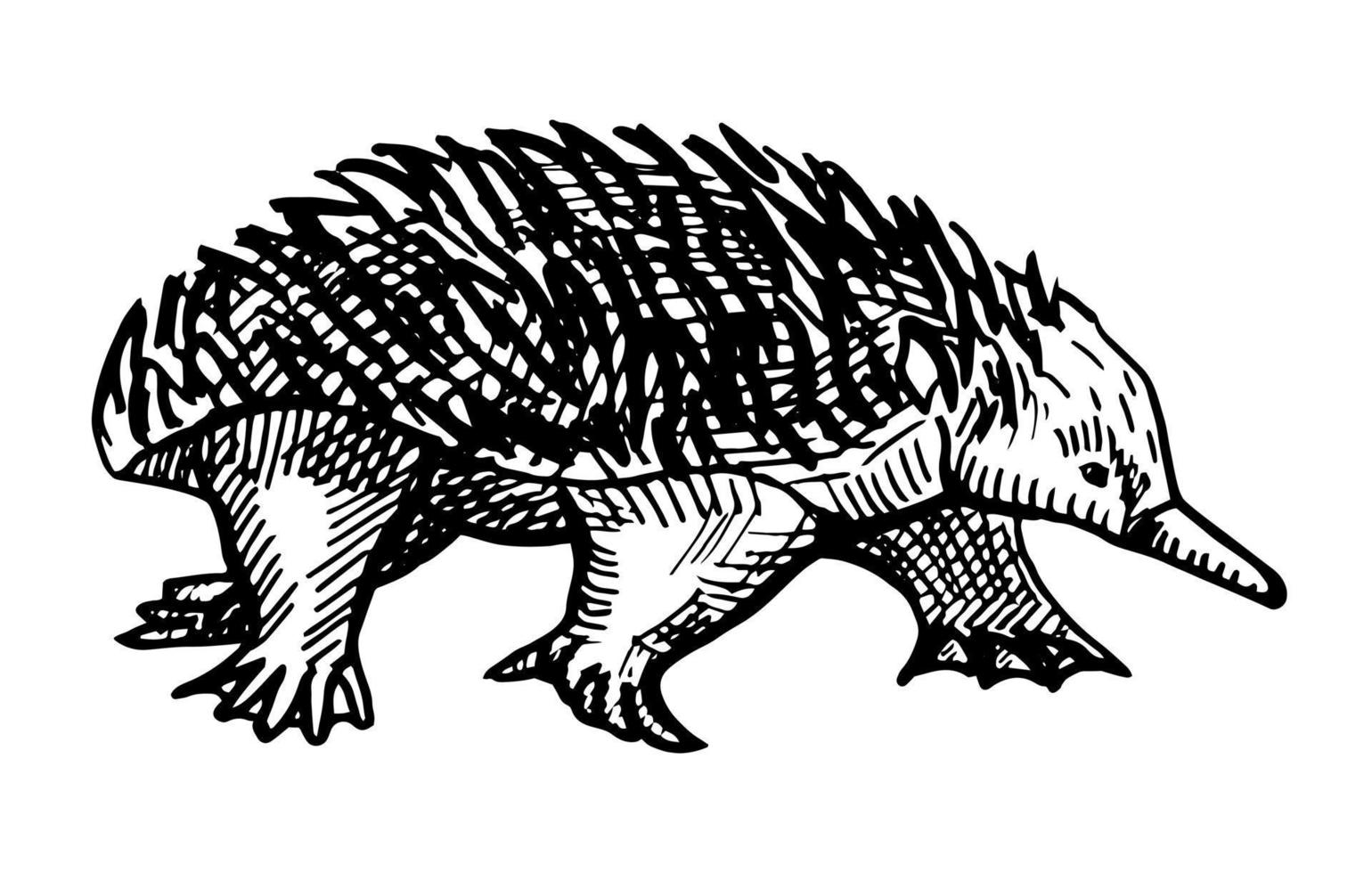This image is a detailed black and white illustration, created with thick black marker lines, depicting an unusual animal. The animal resembles a blend of an anteater and a duck-billed platypus, characterized by a long beak or nose that suggests an adaptation for picking up ants. The drawing has a crude yet artistic style, with dark shadowing achieved using hash marks. The creature is positioned with its bill facing the right side of the frame, and only one eye and ear visible, contributing to its peculiar appearance. Notably, the animal has a back adorned with thick, flared lines resembling quills, akin to a porcupine's. Its legs are stout, ending in large, webbed paws with five toes each, hinting at an aquatic nature. The background is also rendered in black and white, keeping the focus on the intricately detailed and enigmatic creature.